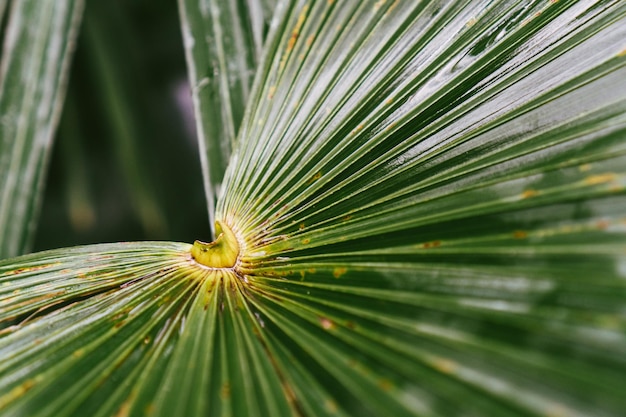This up-close, angled photograph captures the intricate details of a large palm frond. The frond's dark green leaves, featuring a glossy sheen, fan out in textured ridges reminiscent of amphibian toe webbing, seamlessly interconnected with no gaps. In the center of the leaf is a small yellow bulb, possibly a seed that has opened, encircled by a faint white edge. The tip of the leaf angles toward the bottom right of the frame, and the image is slightly out of focus as it extends from the center outward. Specks of brown are visible along the frond's surface, adding to its complex coloration. The rectangular image, wider than it is tall, also features a blurred background filled with similarly textured green leaves, enhancing the sense of depth and focus on the central frond. There are no people, animals, or man-made objects present in this natural, detailed close-up.